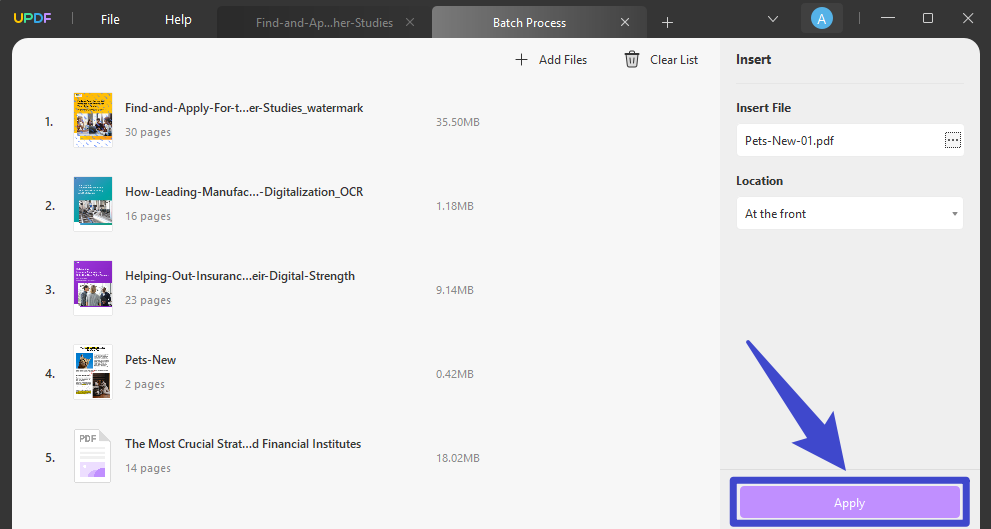The image showcases a software application named UPDF, notable for its colorful branding where each letter of the acronym is represented in a different color: orange (U), green (P), blue (D), and purple (F). 

In the top-left corner of the interface, there are standard menu options: 'File' and 'Help', followed by a search bar which currently has partial text displayed, "find an AP...HER-studies". To the right of the search bar, there is a 'Batch Process' button, indicating the application can handle multiple files simultaneously. Additionally, there is a '+' icon for adding new tabs.

In the top-right corner, a user account icon marked with the initial 'A' is present alongside the typical window controls: minimize, maximize/restore, and close. 

The main section of the interface seems focused on finding and managing PDF files, likely documents or e-books. Search results are displayed below, listing various files with parts of their titles visible, such as "find and apply for T...studies", "watermark", "how leading manufacturer... digitalization", and "OCR, helping out insurance...EIR digital strength, pets-new, the most crucial...D... financial institutes". These files vary in size from 0.42 megabytes to 35 megabytes, and appear to be available for download.